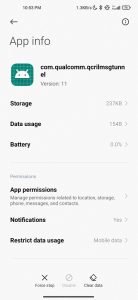The image is a slightly blurry screenshot of an app information screen on a smartphone. Centered at the top, the words "App info" are displayed prominently. To the left of this title is a back arrow that users can tap to return to the previous screen. Also towards the top, typical smartphone status icons are present, including a battery symbol, Bluetooth indicator, a moon icon (likely representing Do Not Disturb mode), and the time, although it is indistinct and only identifiable as sometime in the PM.

Below the "App info" heading, on the left side of the image, there is a familiar green box with an Android symbol. To the right of this icon, the app package name, "com.quacom" followed by some other characters, is shown, indicating the app being referenced. The app version is noted as version 11.

The image further contains sections for app-specific details such as storage, data usage, and battery. However, the exact numbers and details are not discernible due to the blur. Additional options listed below include app permissions, notifications, and restrict data usage.

At the very bottom of the image, there are two icons: an 'X' likely serving as a button for force stopping the app, and another button which possibly reads "Clear data" or something similar. This is a typical app information screen for an Android device, containing all relevant details one might need to manage an app.